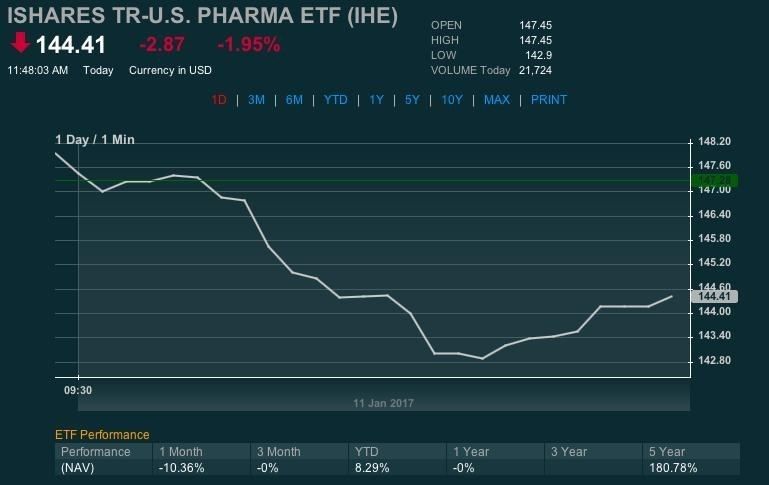This color photograph depicts a computer or laptop screen, oriented horizontally. The focus is on a stock market graph featuring a predominantly black background. The graph displays white text along with additional light blue, green, and red text elements. At the top, the title indicates "iShares TR - U.S. Pharma ETF (IHE)." The graph itself covers a timeframe of "one day/one minute," dated January 11, 2017, and plots time against the dollar value of the stock.

A white line graph illustrates the stock's movements throughout the day. Below the graph, there is a section titled "ETF Performance," featuring columns labeled with various performance timeframes: one month, three months, year to date, one year, three years, and five years. Corresponding performance metrics for each timeframe are listed beneath these headings.